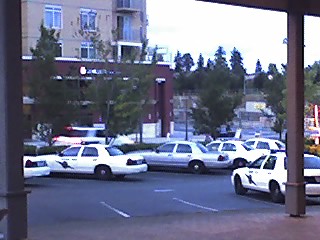The image depicts a somewhat dim and slightly blurry outdoor scene that appears to be taken at a police station. We view the scene from under a brown square-columned overhang, looking out onto a blacktop parking lot marked with white striped spaces. The parking lot features approximately six vehicles, primarily white Ford LTD or Ford Taurus-style sedans adorned with light bars on their roofs and bearing a logo on the side that includes a lightning bolt; however, the text is too small to read clearly. In addition, there is a silver-gray unmarked car, likely used for undercover purposes, parked among them. The background includes a mix of evergreen and deciduous trees under a gloomy sky. To the upper left, a multi-story apartment or tenement building with visible balconies and numerous windows is present. Adjacent to this, a single-story red-brick building, possibly a police garage or fire station, is also visible. In the far right background, yellow-colored vehicles suggestive of construction equipment can be seen partially. The overall image quality is low, with poor lighting contributing to its older, vintage feel.